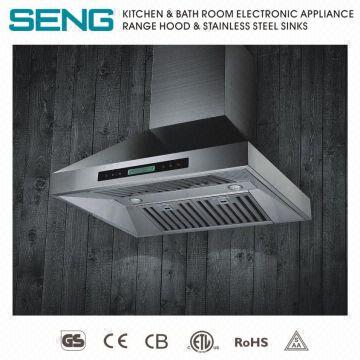This black and white image serves as an advertisement or cover for a kitchen and bathroom electronic appliance, specifically featuring a range hood and stainless steel sinks. At the top, bold text prominently displays 'SENG' in bright blue, followed by the smaller black text reading 'Kitchen and Bathroom Electronic Appliance, Range Hood, and Stainless Steel Sinks.' The central photograph showcases the sleek, stainless steel range hood mounted against a wood-paneled wall. The hood is designed with a large tube that extends downward into a trapezoidal shape with vents. The image focuses solely on the range hood, without revealing any part of the oven or additional kitchen features. At the bottom of the image, several symbols are visible, including G.S.C.E.C.B., E.T.L., Rose, and S.A.A. in a triangle, indicating various certifications and standards. The overall design communicates a sense of modernity and reliability, with 'SENG' standing out in green while the rest of the text and imagery remains monochromatic.